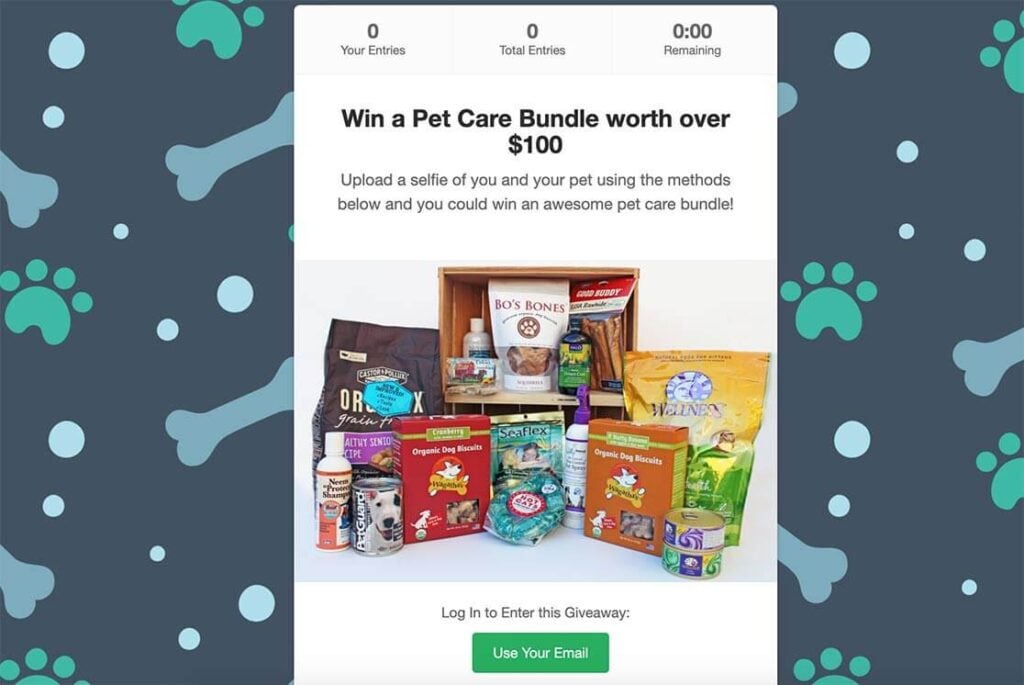This image features a detailed screenshot of a contest web page set within a horizontal frame. The background displays an illustrated design with a gray banner adorned with light gray bone patterns and aqua-colored paw prints interspersed with light blue bubbles on both the left and right sides.

Centrally positioned is a prominent white pop-up box titled "Win a Pet Care Bundle Worth Over $100." This box encourages users to upload a selfie with their pet through the provided methods for a chance to win an impressive pet care bundle. 

At the top of the pop-up box, a very light gray banner presents contest details such as user entries (currently zero), total entries (zero), and a countdown clock indicating the time left.

Beneath this banner, a photograph showcases the enticing pet care bundle, which includes several packages of pet food, treats, supplies, bones, personal care items, itch spray, and various soaps.

Following the image, the text instructs users to log in to participate in the giveaway, with a green button below that reads "Use Your Email."

This vertical pop-up box is strikingly contrasted against the horizontal backdrop, making it the focal point of the image.